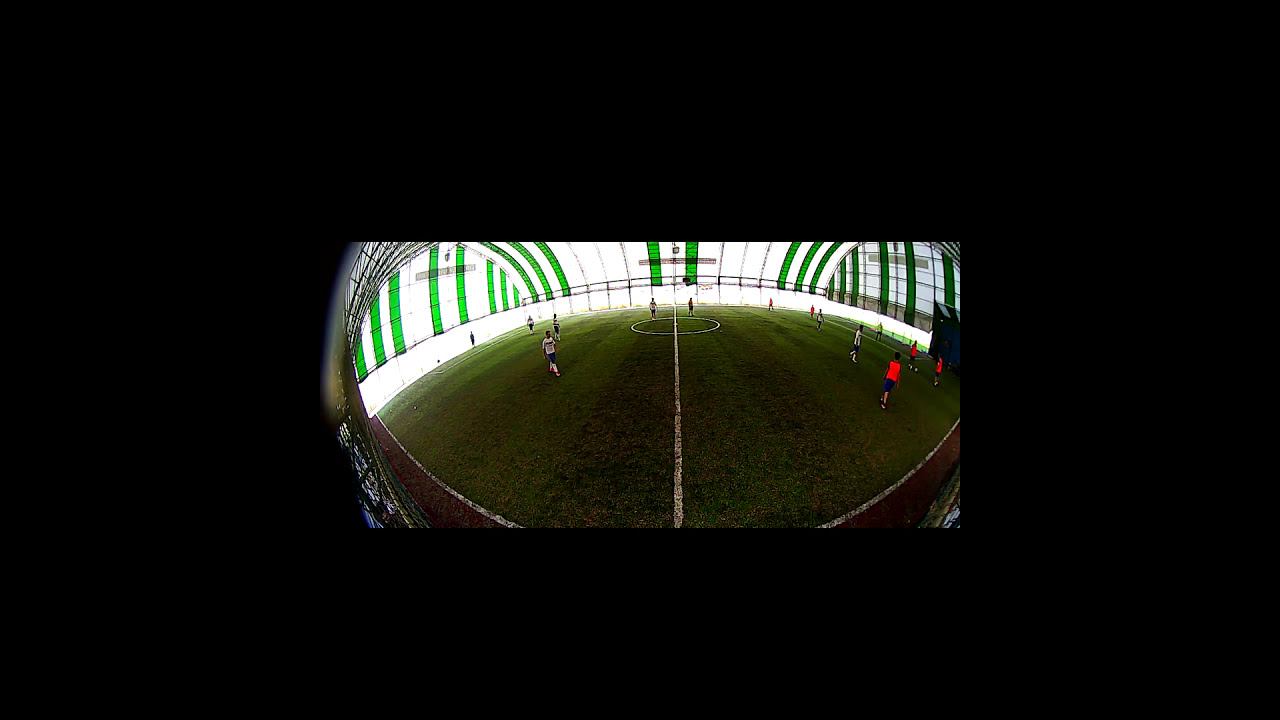The image is a small, color-distorted photograph of a soccer field presented on a large black background, making the photo appear rounded and curved, as if seen through a fish-eye lens. The field itself, a vibrant green with white lines and a central white circle, is unnaturally bowed upwards, giving it an almost volcano-like appearance. Surrounding the field are curved green tiles, and the sides of the stadium appear brightly lit by natural light flooding through, suggesting an indoor arena. 

Two teams of players are visible, wearing distinctive uniforms: one in red shirts and blue shorts, and the other in white shirts and blue shorts. Although the image is small and lacks specific detail, it captures players scattered primarily towards the right side of the field. Despite the indoor appearance suggested by the curved roof, the photograph's clipped edges make it difficult to confirm if the field is completely enclosed. The edges of the image are framed by silver caging and green and white walls, adding to the bewildering spatial perception created by the camera's distortion.